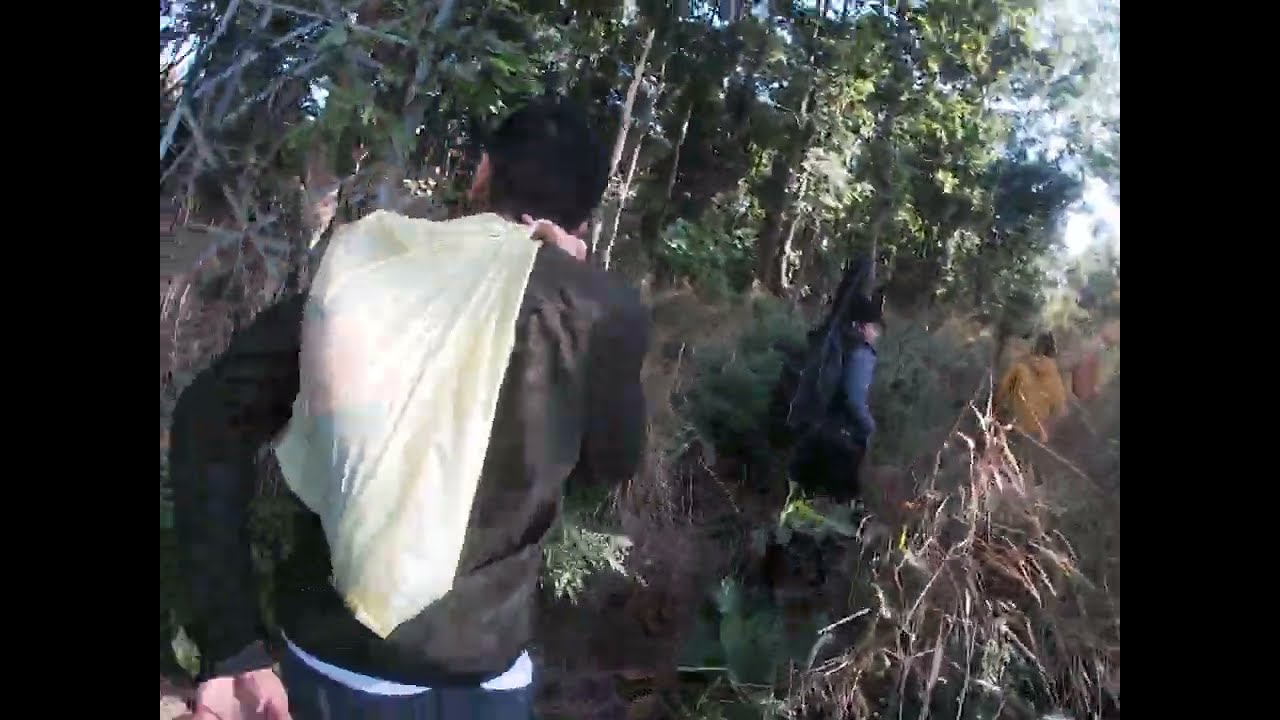A vivid snapshot captures a small group of three individuals on a daytime hike through a dense, verdant forest. The trail is covered in greenery, leaves, and various wild plants sprouting from every direction. Leading the group in the distance is a person in a yellow hooded jacket, casting a stark silhouette against the bright blue sky. Directly in front of the camera, a young man with short dark hair and a dark long-sleeved shirt strides forward, a light-colored bag slung over his back. The trail he treads is flanked by trees, some alive with green leaves and others dead or dry, hinting at the changing season. Between him and the leader in yellow is another individual, partially obscured, wearing a blue shirt with a black vest, also carrying a bag. The unpaved trail appears rugged yet serene, bathed in the warm sunlight filtering through the thick canopy above.